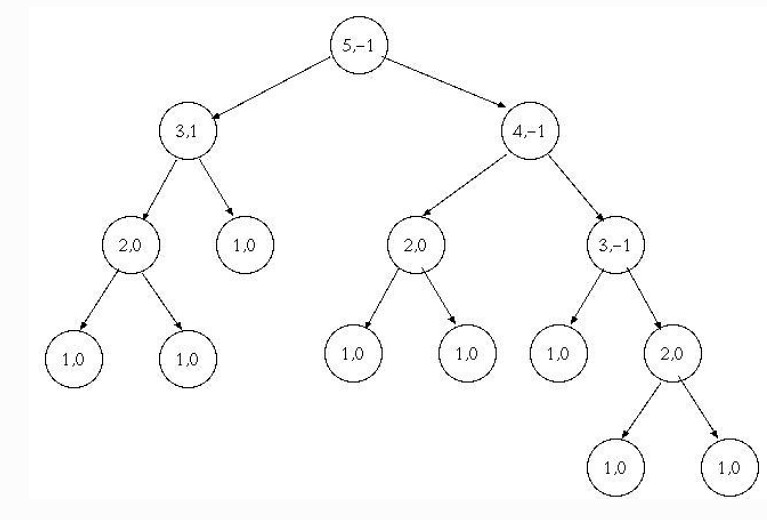The image depicts a flowchart on a white background with black print, seemingly printed out. At the top center, there is a circle labeled "5,-1". An arrow extends to the left, pointing to another circle labeled "3,1". From this "3,1" circle, an arrow extends to the right, marked "1,0". Another arrow extends to the left from the "3,1" circle, labeled "2,0". This "2,0" circle branches further with an arrow to the left, having two "1,0" labels coming out of it sequentially.

Returning to the top circle "5,-1", an arrow points to the right leading to a circle labeled "4,-1". Further to the right, there is another circle labeled "3,-1". To its left is a circle marked "1,0" and to its right, another marked "2,0". The "2,0" circle branches out both right and left, each labeled "1,0".

Returning to circle "4,-1", an arrow extends to the left labeled "2,0". This "2,0" circle subsequently splits into two separate arrows both marked "1,0".